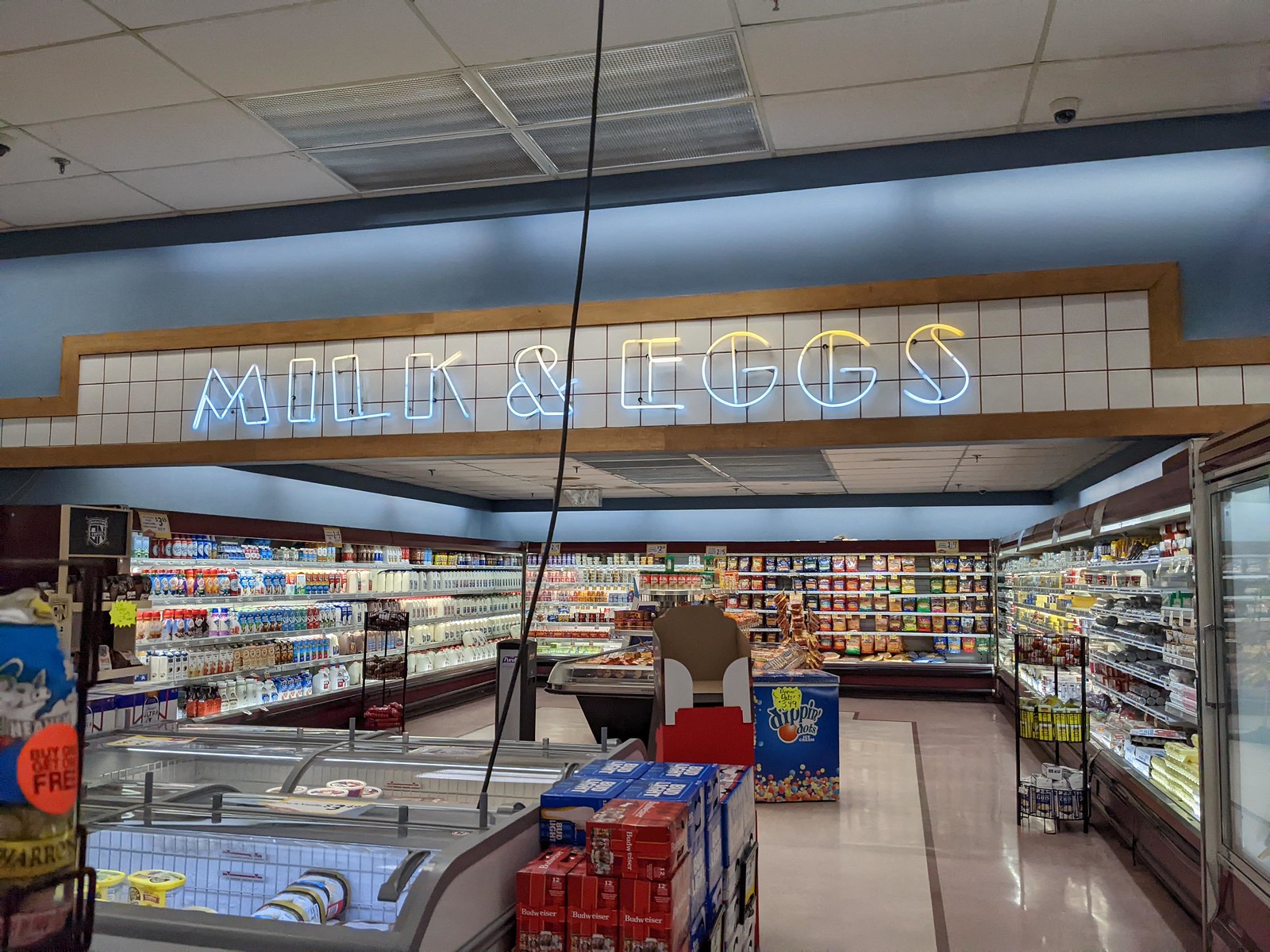The image captures a high-angle view of the interior of a grocery store. From this elevated perspective, the store's expansive layout is clearly visible, showcasing an efficiently organized and brightly lit space. Dominating the scene is a charming alcove section that houses its own small enclave, signified by a prominent sign overhead. The sign, emblazoned in all-caps and illuminated by blue and white neon lights, reads "MILK AND EGGS." 

The shelves within this section are brimming with a variety of dairy products, meticulously arranged to create an appealing display. To the right, there's an extensive assortment of egg cartons, each neatly stacked and offering different varieties. The left side is dedicated to an impressive collection of milk, with bottles and cartons of various sizes and brands. Nestled between these sections, the central area likely features other dairy products, possibly including an array of yogurts and cheeses, contributing to the colorful and well-stocked appearance of the store. The overall atmosphere is one of abundance and careful organization, inviting shoppers to explore the diverse offerings.